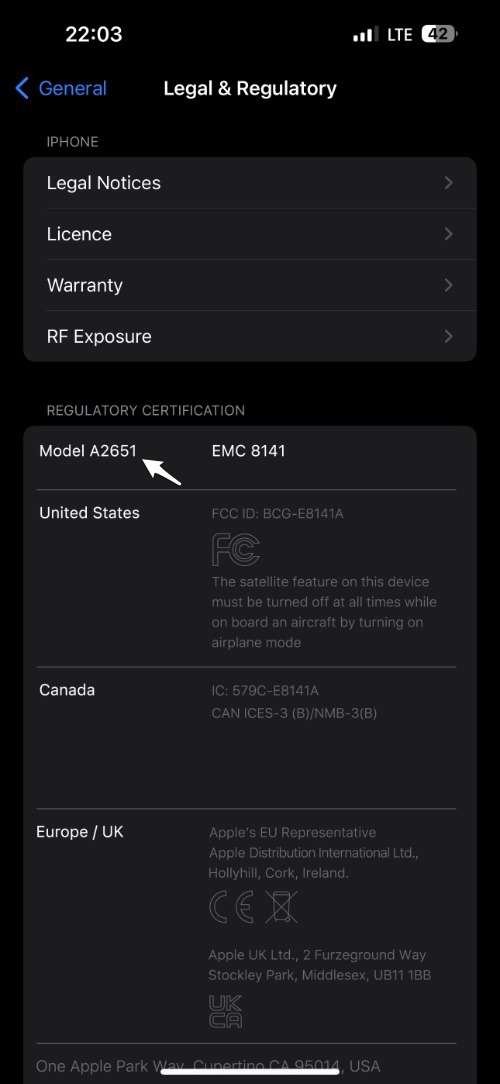This screenshot from a mobile phone, displayed in dark mode, features a black background with contrasting white and purple text. 

- **Top of the Screen:**
  - **Left Corner:** The time is displayed as '22:03' in white font.
  - **Right Corner:** The mobile signal strength shows three out of four bars, with 'LTE' indicating the network type and the battery level reading '42%'.

- **Middle to Lower Section of the Screen:**
  - **Top Bar:** The label 'Legal and Regulatory' is shown in the bottom center of the screen. To its left, 'General' in purple font is accompanied by a left-pointing arrow.
  - **Below the Top Bar:** The word 'iPhone' appears in gray font.
  - **Options Menu:** Four gray rectangles list selectable options: 
    1. 'Legal Notice'
    2. 'License'
    3. 'Warranty'
    4. 'RF Exposure'
  - **Post-Options Section:** Below the options menu, 'Regulatory Certification' appears in gray font, followed by a larger gray rectangle.

- **Within the Large Gray Rectangle:**
  - The upper left corner reads 'Model A2651' with a small right-pointing arrow next to it.
  - To the right, it states 'EMC 8141'.
  - Below this, a line separates another piece of text that reads 'United States FCC ID BCG-E8141A'.